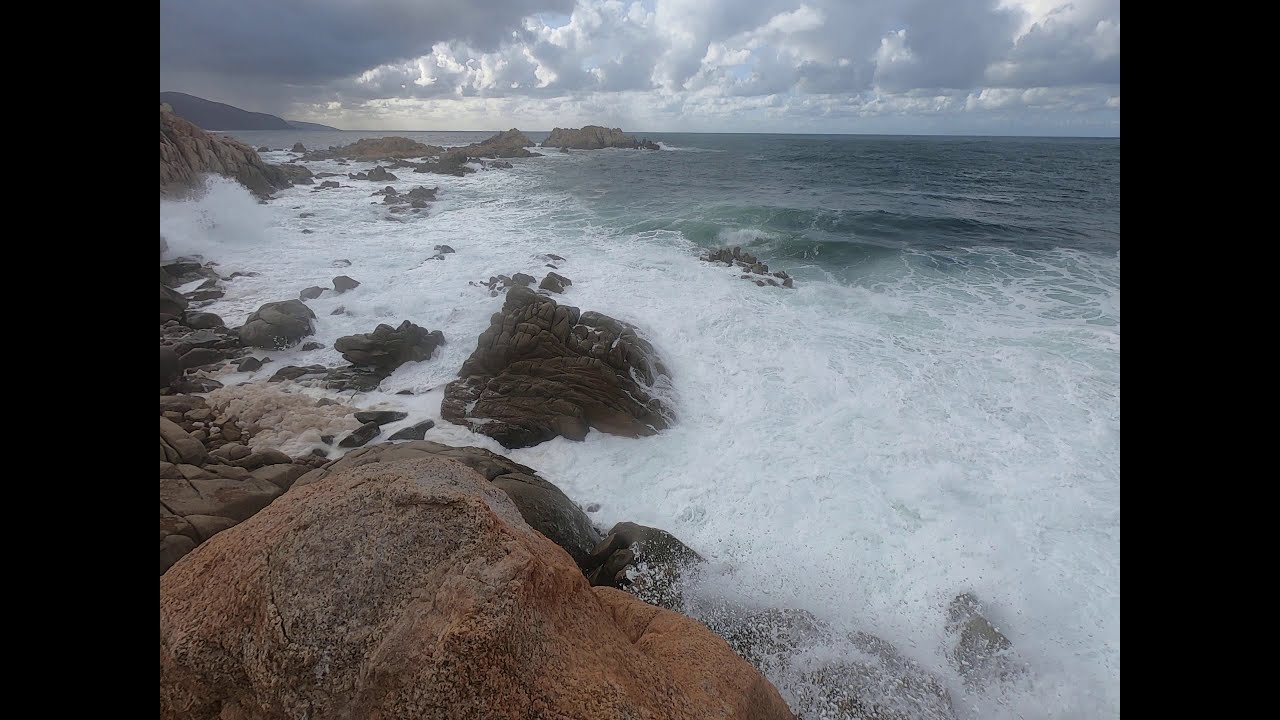The image showcases a dramatic rocky beachside under a sky filled with white and grey clouds, with no visible sun. The turbulent ocean waves, mostly blue and green, turn into white froth as they crash against the shoreline. The bottom left corner of the image is dominated by various dark-colored rocks and a small cliffside. Water droplets from splashing waves are visible in the bottom right corner. In the far distance, towards the top left of the image, a large hill or mountain is discernible. The horizon line splits the ocean from the sky, adding depth to the scene. The image is framed with black bars on both the left and right sides, enhancing its moody atmosphere.